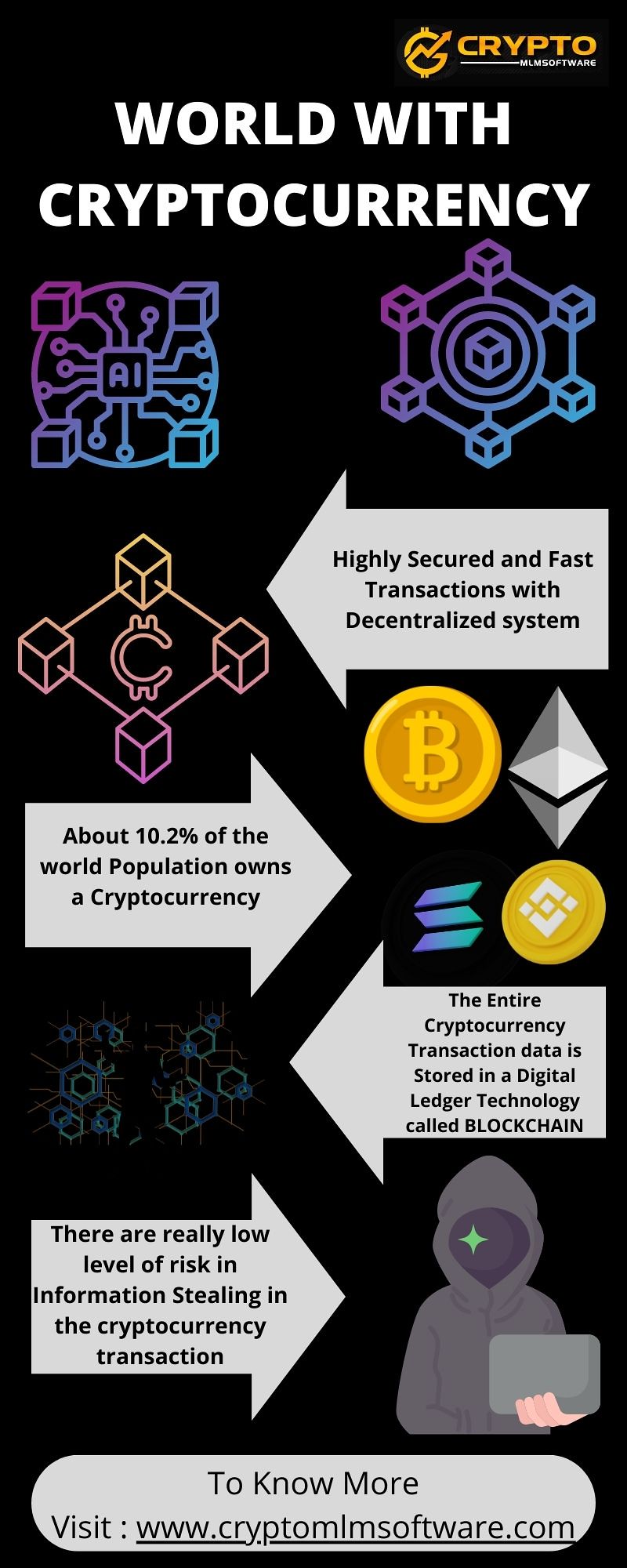This vertical rectangular banner, set against a black background, promotes cryptocurrency education and adoption. At the top right corner, orange letters spell "crypto" next to a logo resembling a stock market icon with a lightning bolt and upward arrow. Below, in bold white text spanning the width, it reads "world with cryptocurrency." The design includes purple, pink, and orange geometric and digital elements: one symbolizing artificial intelligence with an "AI" center and outward-reaching lines, another depicting interconnected cubes, representing blockchain, and a "C" in the middle of a network indicating cryptocurrency. 

Several arrows point to explanatory sections: a white arrow highlights "highly secured and fast transactions with decentralized systems," directing attention to interconnected squares. Another arrow informs that "about 10.2% of the world population owns a cryptocurrency," accompanied by Bitcoin and other cryptocurrency logos. Further text explains, "the entire cryptocurrency transaction data is stored in a digital ledger technology called blockchain," targeting blockchain symbols. Lastly, it notes "there are really low levels of risk and information stealing in cryptocurrency transactions," illustrated by a hooded figure with a green sparkle holding a device. For further information, viewers are directed to visit www.cryptoMLMsoftware.com.